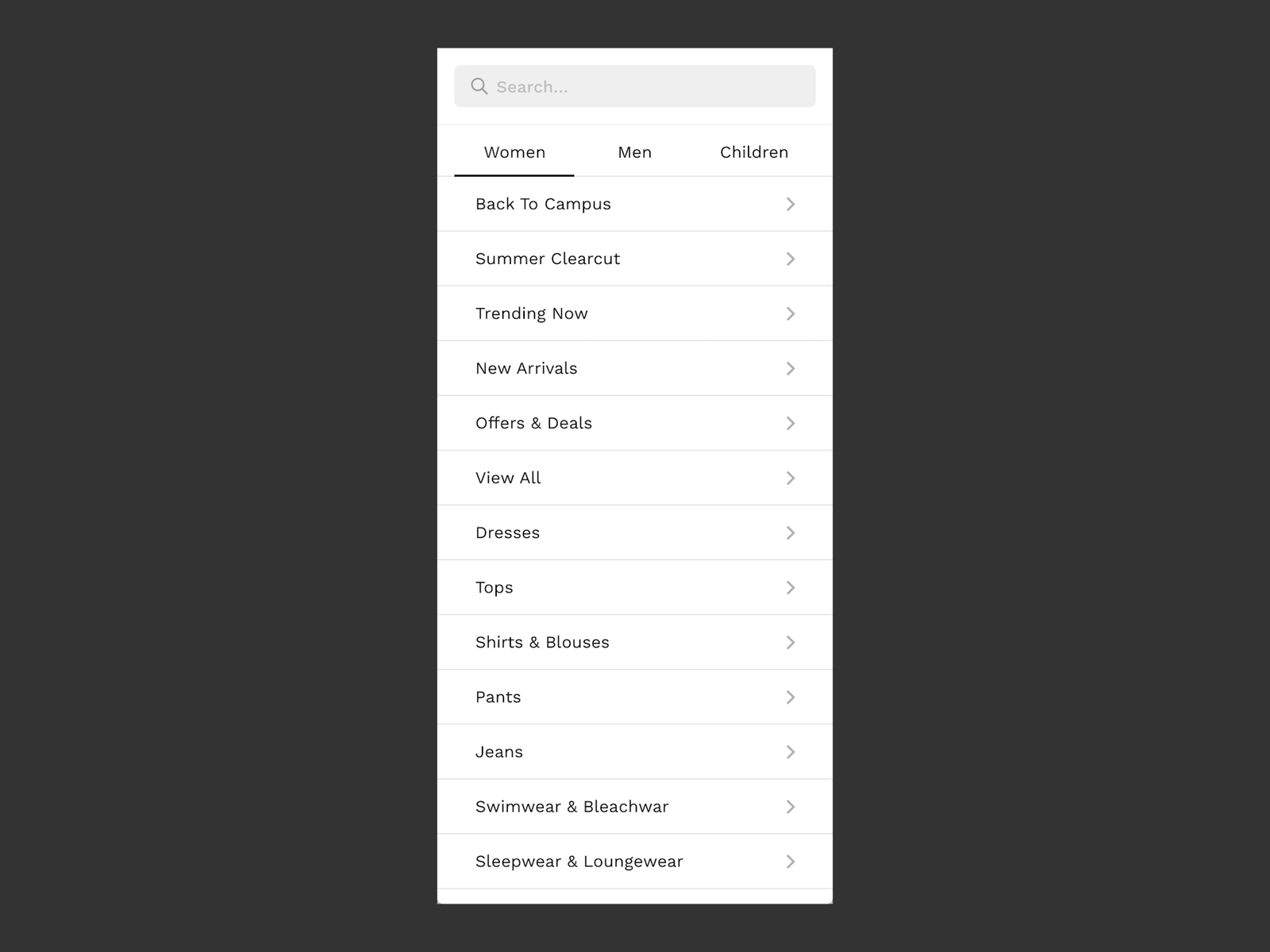The image features a stark, minimalist design with a large black rectangle serving as the background. Centrally placed within this black expanse is a taller, thinner white rectangle, reminiscent of a smartphone screen.

At the top of the white rectangle, there is a gray search bar featuring a magnifying glass icon accompanied by the placeholder text "Search..." in gray letters.

Beneath the search bar, there is a horizontal menu with categories labeled in black print: "Women," "Men," and "Children." The "Women" category is underlined with a black line, indicating it is currently selected.

The main content area, focused on women's items, is divided into multiple sections. Each section's title is in black text, aligned to the left, with a small gray arrow (resembling a sideways "V") pointing to the right. These sections are separated by faint gray lines. The categories listed from top to bottom include: "Back to Campus," "Summer Clearance," "Trending Now," "New Arrivals," "Offers and Deals," "View All," "Dresses," "Tops," "Shirts and Blouses," "Pants," "Jeans," "Swimwear," and "Loungewear."